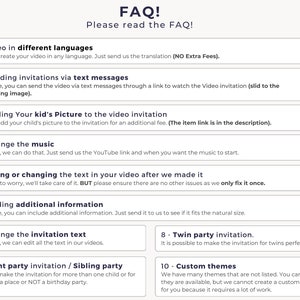In this image, there is a structured FAQ (Frequently Asked Questions) section, predominantly featuring text with specific formatting and categories. At the very top center, the title "FAQ!" is prominently displayed in dark blue font, making it immediately noticeable. Directly beneath this title, in slightly smaller font and lighter gray background, is a prompt urging readers to "please read the FAQ."

A horizontal line, possibly in the same dark blue as the title, serves as a divider, segmenting the FAQ content into distinct sections. Despite being partially cut off on the left side, the first category mentions "No extra fees" and lists different languages. 

The second category discusses "invitations via text messages," explaining that a video invitation link can be sent via text. The third category outlines how to include "your kid's picture" in the video invitation for an additional fee, with further details about the item link provided in the description.

Positioned in the middle of the image, the fourth category addresses music customization options, indicating users can send a YouTube link specifying when they want the music to start in the invitation.

Further down, there are four additional sections covering various topics such as "Changing the text in the video," "Additional information," "The invitation text," and "Party invitation," thereby offering comprehensive guidance on modifying and personalizing the video invitations.